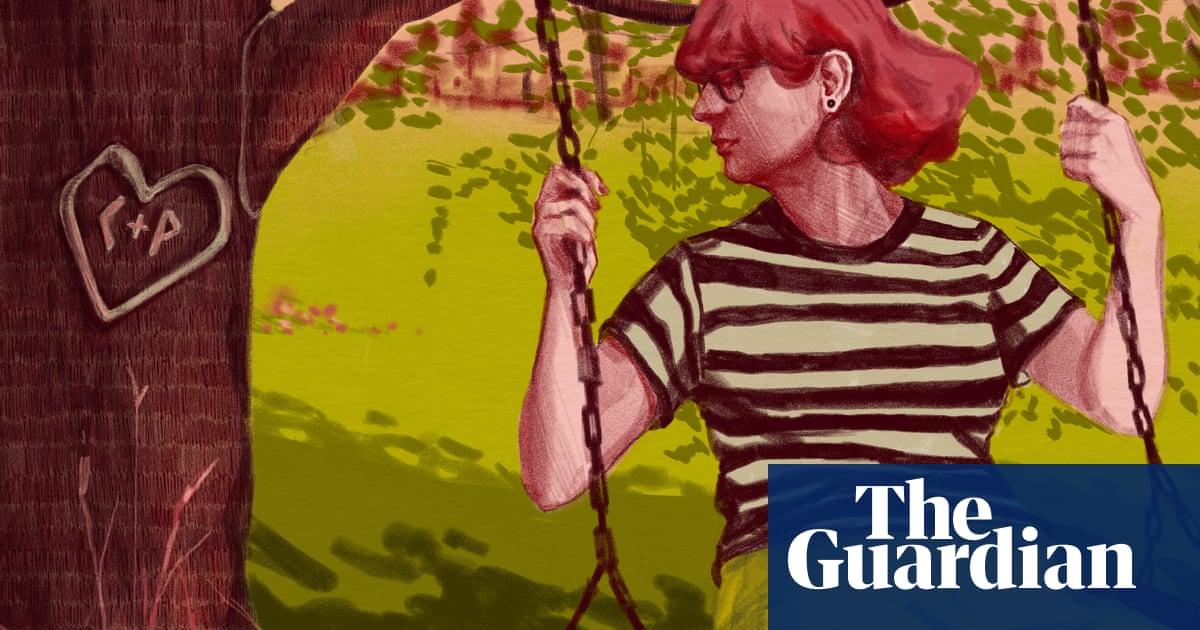The image depicts a detailed painting of a young woman with red hair, styled with bangs and slightly flipping up at the back, swinging on a swing suspended from a tree by metallic chains. Her head is tilted to the left, and she wears glasses along with a black and white striped t-shirt. The swing's base is not visible, but her hands grip the chains firmly. The tree to her left has a brown trunk adorned with a carved heart, inside which the initials "C + P" are inscribed. The background features a grassy ground and some leaves. On the bottom right corner of the image, a blue rectangular box with white text reads "The Guardian," suggesting it might be a banner or featured graphic for the online publication.